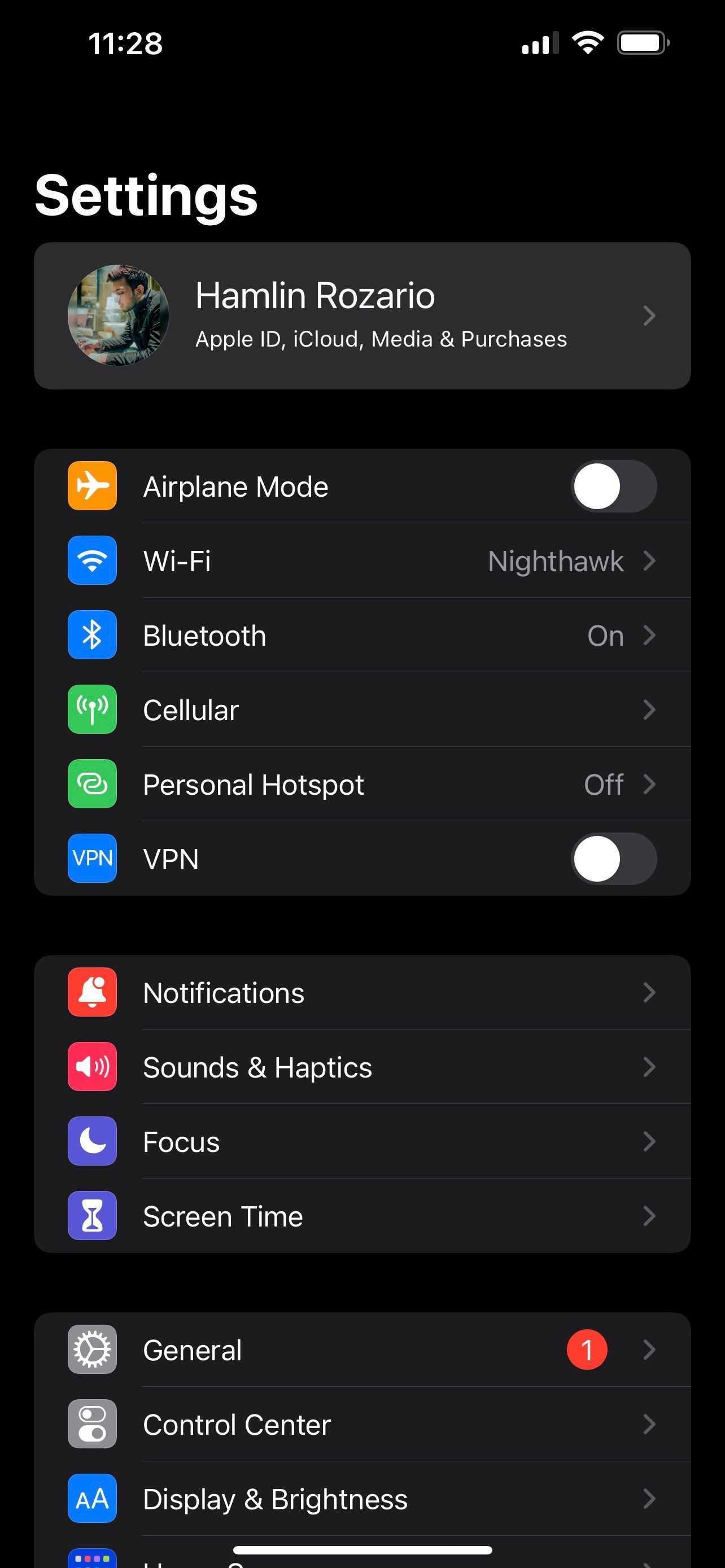The image showcases the "Settings" page on an iPhone. The background is entirely black, providing a stark contrast to the vibrant icons and text. At the top of the screen, the user's information is prominently displayed, which includes the name "Hamlin Rosario" along with the tags "Apple ID, iCloud, Media & Purchases." A small profile picture of a man appears to the left of this information.

Below this section, a list of settings options is aligned vertically along the left side:

1. **Airplane Mode**: Represented by an orange box with a white airplane icon. The slider next to it indicates that airplane mode is currently turned off.
2. **Wi-Fi**: Displayed with a blue Wi-Fi symbol, showing a connection to a network named "Nighthawk."
3. **Bluetooth**: Illustrated by a symbol resembling a pair of intertwined AirPods, marked as "On."
4. **Cellular**: Indicated by a right-pointing arrow, suggesting more options are available upon selection.
5. **Personal Hotspot**: Shown with a green icon next to it, indicating that the personal hotspot feature is turned off.
6. **VPN**: Represented by a box with "VPN" inside it, with the corresponding slider showing that the VPN is off.
7. **Notifications**, **Sounds & Haptics**, **Focus**, **Screen Time**, and **Control Center**: These settings are listed without additional icons or markers.
8. **General**: Notably, this section has a red circle with the number "1" in it, signaling a pending notification.
9. **Display & Brightness**: Listed among the various options available within the settings menu.

Overall, the organized layout and visual indicators provide a comprehensive overview of the phone's current settings.